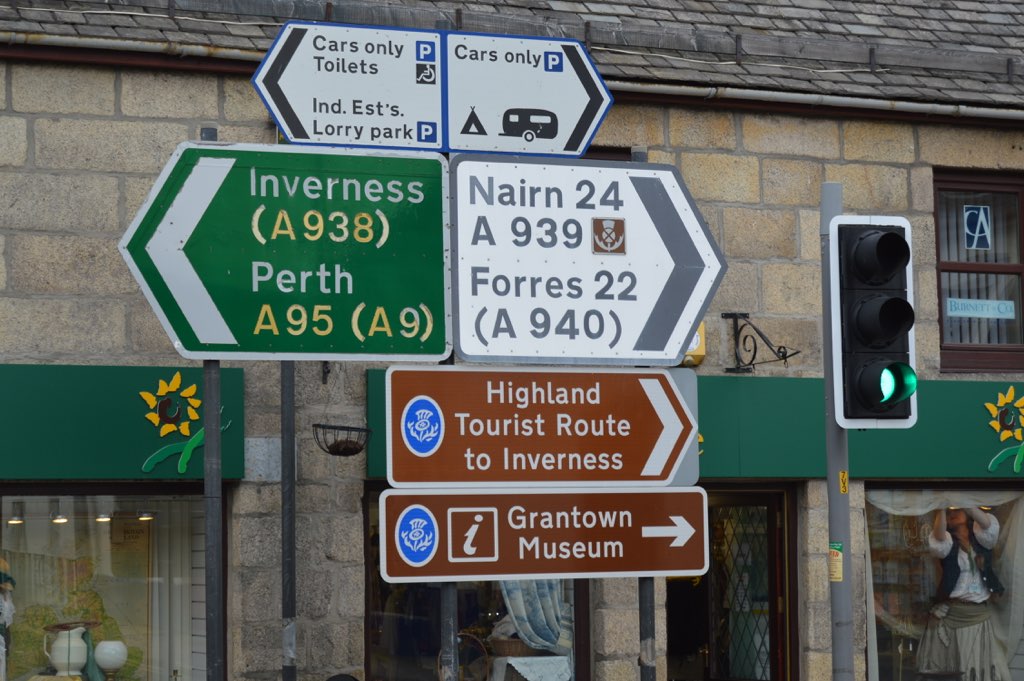The image depicts a cluster of street signs mounted next to a stoplight, which is currently green, in front of a small shopping district characterized by an older brick building. The signs detail various directions and resources: "Cars Only, Toilets, End Est Lorry Park" with arrows pointing left, and "Cars Only," featuring a camper and a tent icon, pointing right. Below them are larger signs indicating routes and distances—pointing left to "Inverness (A938)" and "Perth (A95, A9)," and pointing right to "Nairn 24 (A939)" and "Forres 22 (A940)." Further down, two additional signs, both with right-pointing arrows, direct to "Highland Tourist Route to Inverness" and "Grantown Museum." The background reveals multiple stores with visible windows, including a woman decorating the interior of one store, and the daylight exterior provides bright and clear visibility.